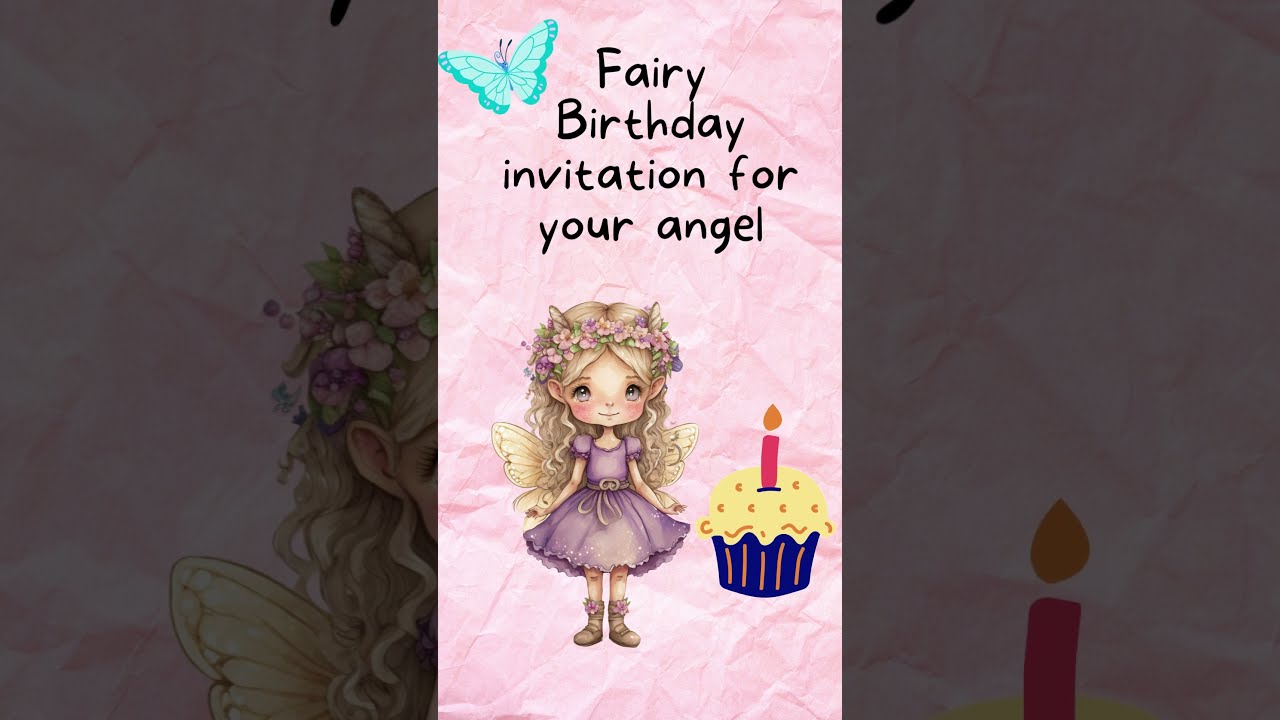The image is a whimsical birthday invitation with a predominantly pink background resembling crumpled paper. At the top, in a handwritten black font, it reads, "Fairy birthday invitation for your angel." Adjacent to this text is a light blue butterfly graphic. Below, there is a charming illustration of a fairy with blonde hair, blushing cheeks, and a pink flower crown. She wears a purple dress with butterfly-like wings and brown boots. To her right, a contrasting art style showcases a clipart cupcake with yellow frosting, a blue wrapper, and a single red candle with an orange flame.